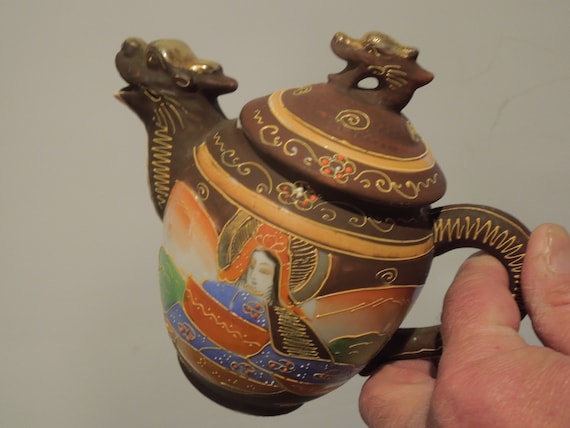The image features a small, ornate antique teapot with a distinctly ancient Chinese aesthetic. The teapot, held at an angle by a person’s left hand coming from the bottom right corner, stands against a gray background. It is crafted from a dark brown clay and features a spout shaped like an open-mouthed dragon head, hinting at its age and cultural origin. The lid, also adorned with a dragon’s head, serves as a handle.

The teapot is elaborately decorated with intricate golden piping and designs that traverse its surface. On the side of the teapot, a detailed painting depicts a woman in a blue robe with an orange headdress, engaging in what appears to be food preparation. This scene and the teapot's dragon motifs highlight the blend of functionality and artistic expression typical of antique Chinese pottery. The craftsmanship and detailed ornamentation make this teapot not only a utilitarian object but also a piece of historical artwork.